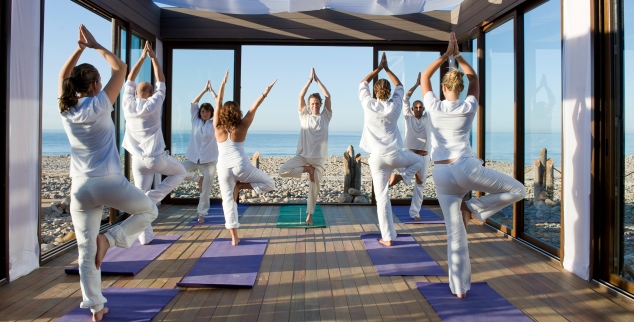This photograph captures a serene yoga session set inside a glass building with large windows on three sides, offering a stunning view of a pebble beach and an expansive body of water. The wooden floor surface enhances the natural and tranquil ambiance of the space. The scene features five participants, dressed uniformly in white tops and white slacks, engaging in a yoga pose where they balance on one foot with the other foot placed on their inner thigh, and their arms raised above their heads. There are three female participants and two male participants, all standing on purple yoga mats. Leading the session are three instructors—two men and one woman. Notably, while the instructors also mostly use purple mats, the male instructor in the middle stands on a distinctive green mat, drawing the eye. The participants face away from the camera, focusing intently on the calming instructions from their teachers who face the camera. This meticulously staged image, possibly for an advertisement or promotional material, elegantly portrays the harmony and dedication inherent in practicing yoga within such a picturesque and peaceful environment.